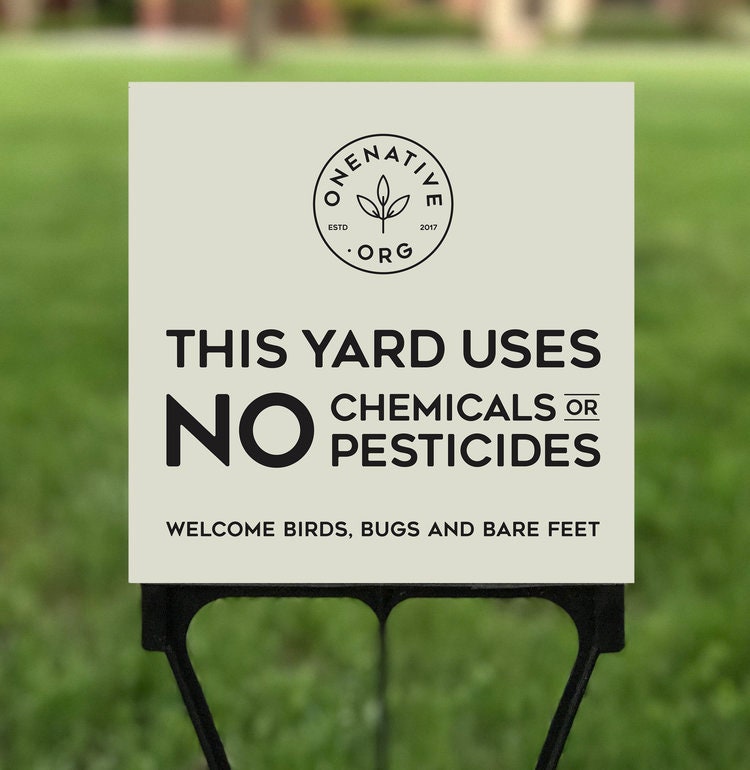The photograph features a white, square yard sign with prominent black text. The most eye-catching part of the sign is the bold, large "NO," indicating that the yard uses no chemicals or pesticides. Below this, the message continues in smaller text: "Welcome birds, bugs, and bare feet." Positioned at the top center of the sign is a circular logo featuring a three-leaf plant icon, with the text "OneNative.org" and "Established 2017" wrapping around it. The sign is mounted on a three-spoke black frame, staked into an out-of-focus grassy yard in the background.